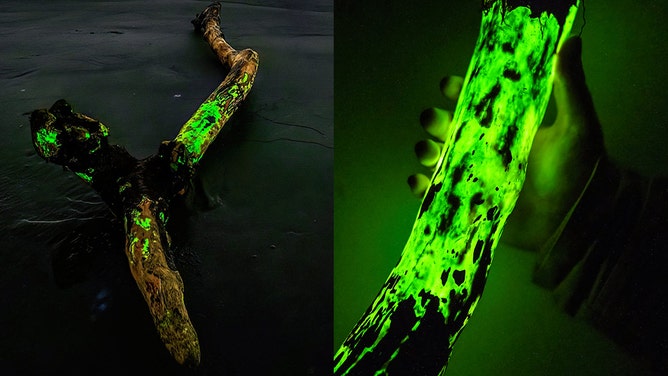The image is a juxtaposition of two photographs depicting an eerie scene revolving around a gnarled tree branch covered in phosphorescent green slime. On the left side, the main image features the tree branch, which appears to be lying on a beach. The branch is encrusted with glowing green slime and bears a peculiar large black shape in its center, extending towards the top left. This enigmatic shape is adorned with gold stripes and also smeared with the luminous green slime, presenting an almost otherworldly appearance. The right side of the composite showcases a close-up of the glowing green slime in a darker setting, further accentuating its luminescence. Adding to the intrigue, a man's hand, clad in a long-sleeve shirt, is spotted holding what seems to be a detached piece of the phosphorescent branch, emphasizing the tactile, ethereal quality of the glowing substance. The entire composition is bathed in a greenish hue, contributing to the mysterious and somewhat unsettling atmosphere.